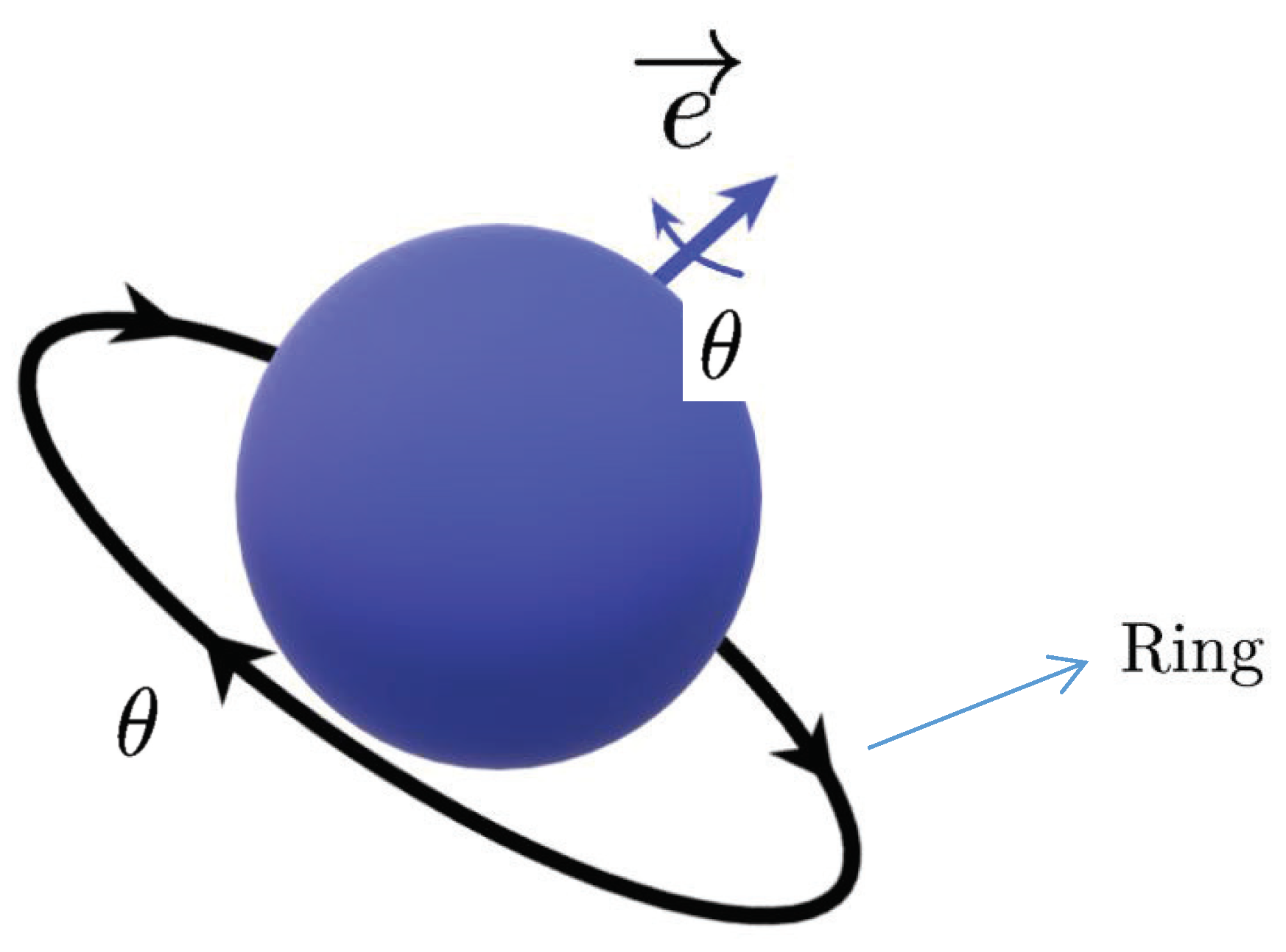In the image, there is a blue orb set against a white background. At the base of the orb, a black line with arrows indicating a clockwise spin extends diagonally from the top left to the bottom right. Around the orb, a black circular ring is marked with black arrows, also indicating a clockwise direction. From the two o'clock position on the blue orb, a blue arrow points upwards and to the top right, beneath which is a black zero on a white background. Above this blue arrow is a black 'E' with a black arrow pointing to the right. As you move down towards the four o'clock position, there is black text labeling a blue line extending from the central black line as "RING." The bottom edge of the orb appears slightly darker. Additionally, there are purple and green arrows surrounding the orb, including a purple arrow pointing out to the top left. Finally, another symbol of a black zero with a dash appears both near the ring and at the top of the orb.